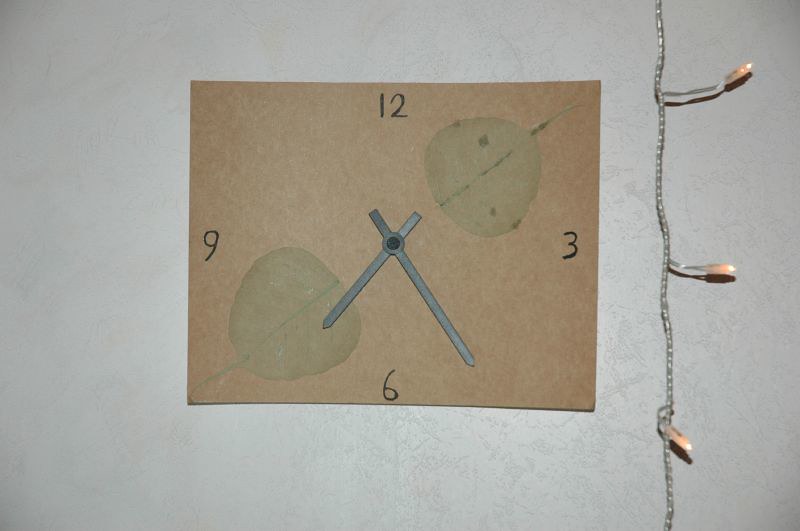This is a photograph of a hand-drawn clock, made from a brown piece of cardboard or construction paper, prominently featuring the numbers 12, 3, 6, and 9 written in black marker at their respective positions. The clock hands, which appear to be crafted from gray construction paper, are set to approximately 7:25. The clock is mounted on a white wall, although parts of the background appear gray and stucco-like. There are visible blue stains on two spots of the cardboard face. Along the right side of the image, a wire with three white LED lights, resembling Christmas lights, hangs down.